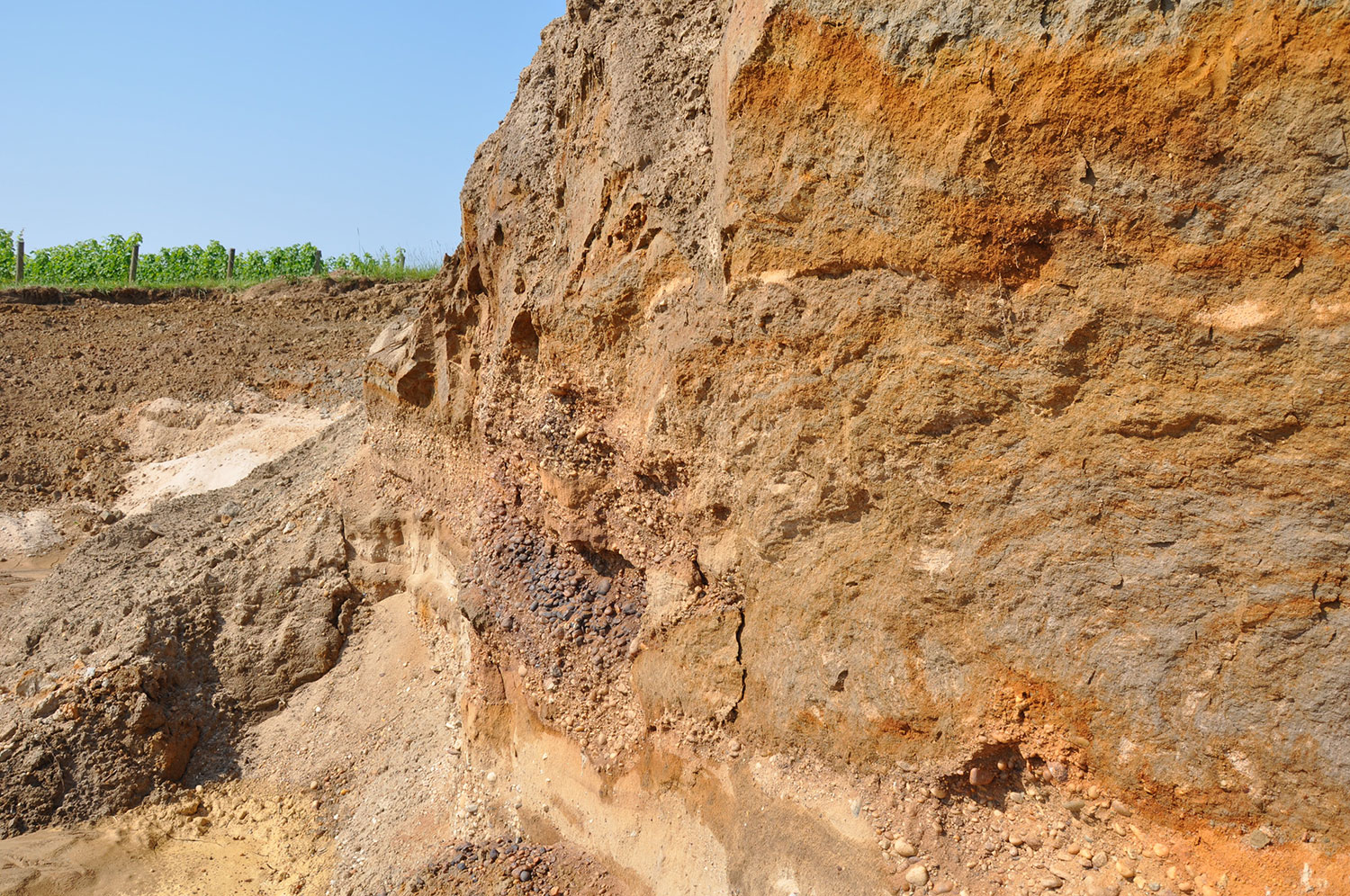This image captures a striking scene of an excavation site, dominated by a vast, orange-brown rock formation on the right-hand side. The rock formation stretches from the bottom to the top of the photograph, appearing as if it has been systematically dug away, exposing layers of dirt, clay, and rock in hues of orange, brown, and red. The left side of the image opens up to reveal a patch of dirt and a neatly cultivated field or orchard, with rows of green plants growing between wooden posts. Above this, in the top left corner, the blue sky peeks through, clear and cloudless. The earthy colors of the rock contrast vividly with the verdant green of the plants and the soft blue of the sky, creating a dynamic and visually engaging composition. The setting suggests an outdoor, agricultural, or archaeological site on a bright, clear day.